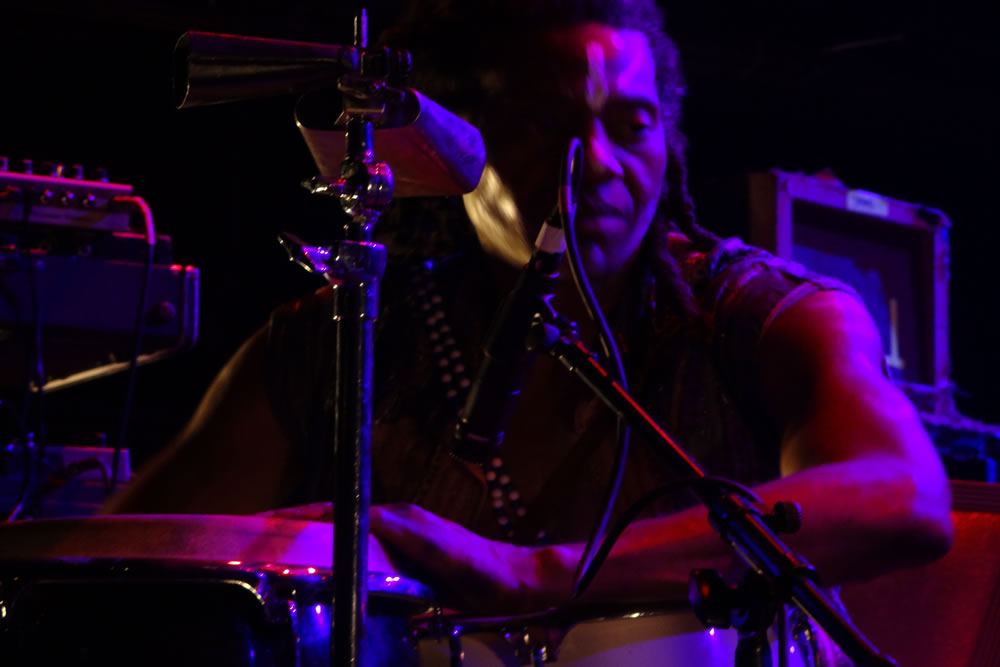This evocative color photograph captures an African descent drummer immersed in a moment of intense performance, possibly at a darkly lit indoor concert or club. Bathed in a purplish hue, the scene showcases his intricate percussion setup in the foreground. A silver metal bar with a cowbell is placed to the left, positioned in front of a partly visible keyboard. To the right stands a black microphone with a trailing cord, while a bongo drum with a striking red top can be seen on the lower left. The drummer, donning a vest and sporting long black hair, is adorned with a white slash of makeup on his forehead, adding to his vivid presence. His body faces forward, though his face is slightly turned to the side. His left hand rests on the higher bongo drum, with another, a white drum, positioned just below it. The backdrop remains inky black, accented by blue stage equipment to the right. The spatial arrangement and the dark, moody atmosphere suggest an intimate, night-time setting where every detail contributes to an immersive auditory and visual experience.